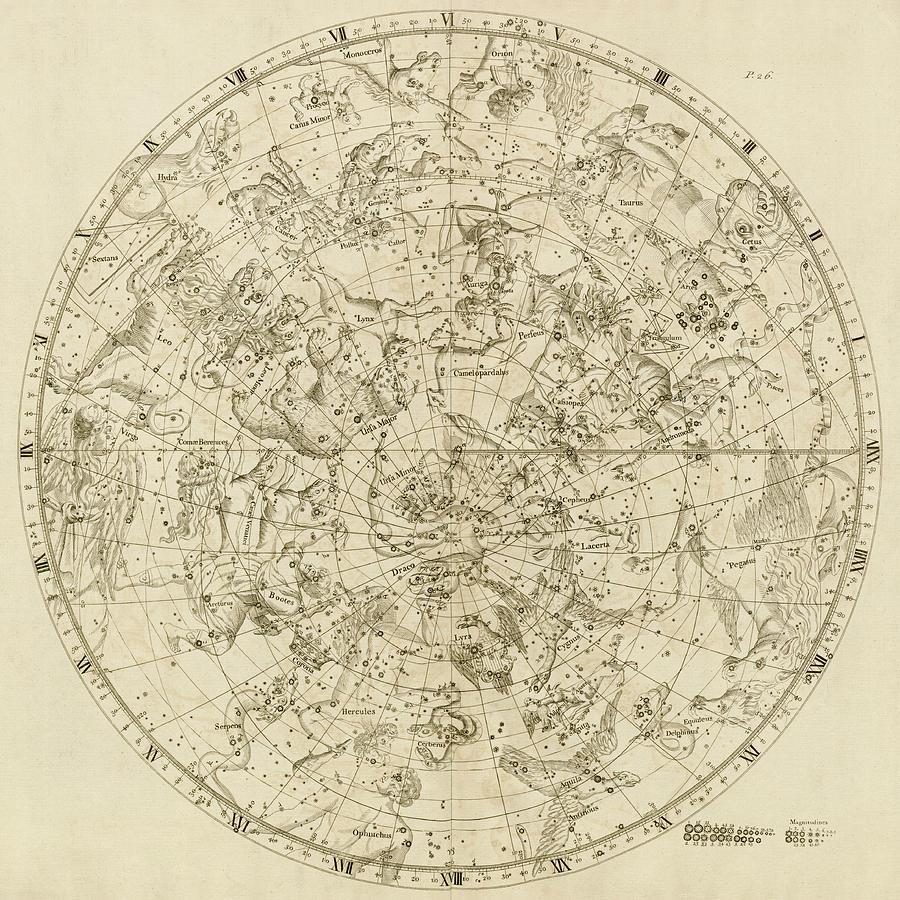The image depicts a vintage constellation map with a faded peach background, illustrated in the form of a globe. Around the outer edges of the globe, various Roman numerals are arranged counterclockwise, starting at four o'clock with "I" and progressing upwards, indicating positions or times. The map is richly detailed with star constellations represented by both dots and intricate lines. In the center, detailed sketches of mythical beings and animals are used to represent the constellations. Among these, you can see specific illustrations labelled as Pegasus, Ursa Major, Hydra, Canis Minor, and Monoceros. Additional names and constellations like Hercules, Draco, and Taurus are also included, along with potentially fading Latin names. The artwork evokes a classical sense of mythology, complete with gods and creatures from ancient beliefs.